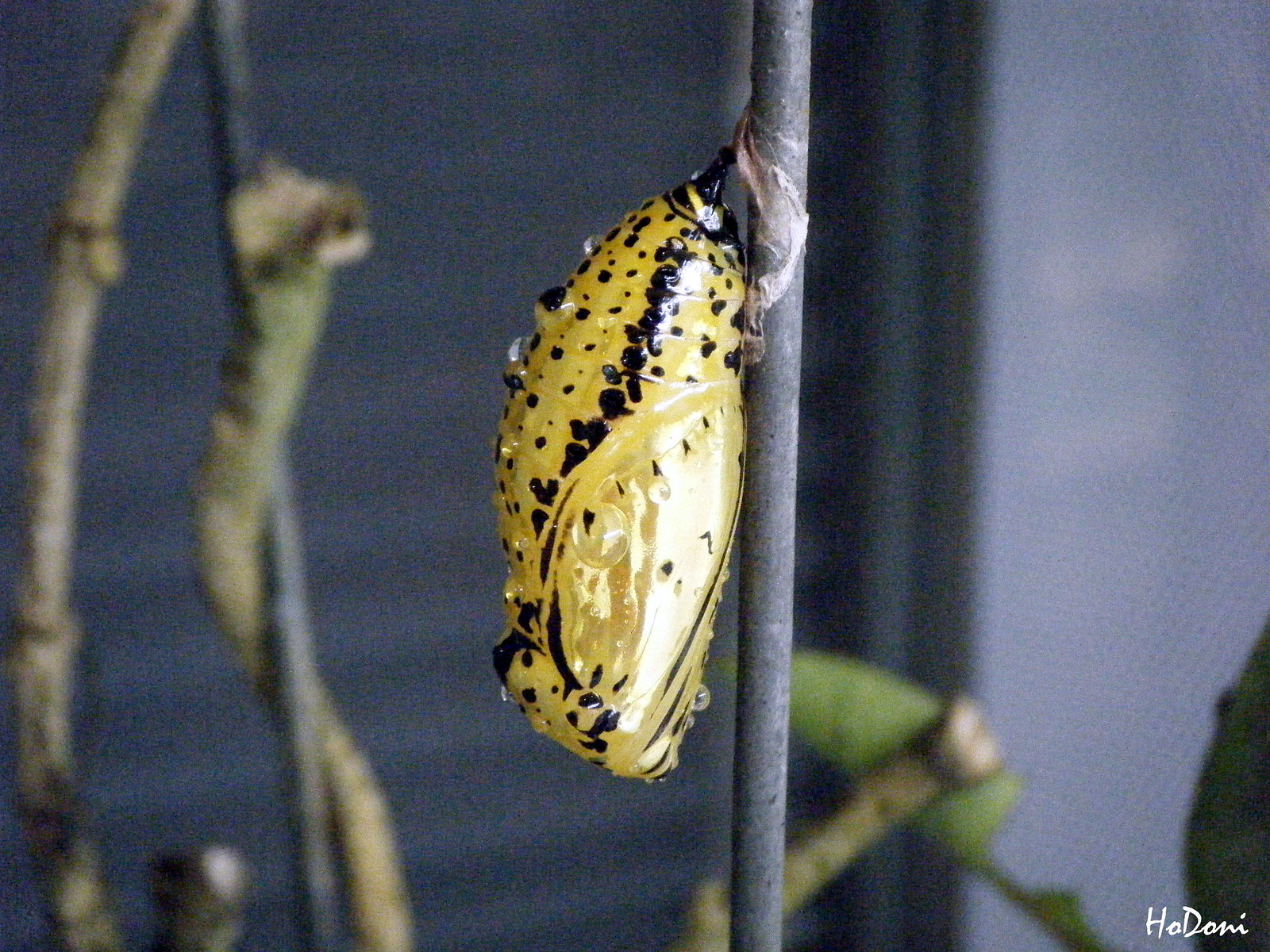This intricate photograph captures a vivid close-up of a chrysalis, likely belonging to a butterfly or moth, attached to a slender metal rod, which runs vertically near the center-right of the image. The chrysalis is predominantly yellow with various black spots and a few white spots higher up. Notably, it has a distinct black mark resembling a beak at its tip that seems to touch the rod. The background of the image is artistically blurred, enhancing the focus on the chrysalis. On the right side, the backdrop transitions into a lilac hue, merging into black, and then navy blue as one moves leftward. To the far left, a slightly curved brown tree branch extends from the top to the bottom of the photo, accompanied by a straight branch with what appears to be a curving leaf encircling it. The setting includes subtle hints of greenery. This outdoor scene is illuminated by daylight, though the exact time cannot be discerned due to the lack of visible shadows. Notably, the image bears the signature "HODENI," with both the 'H' and the 'D' capitalized, placed at the bottom of the photograph.